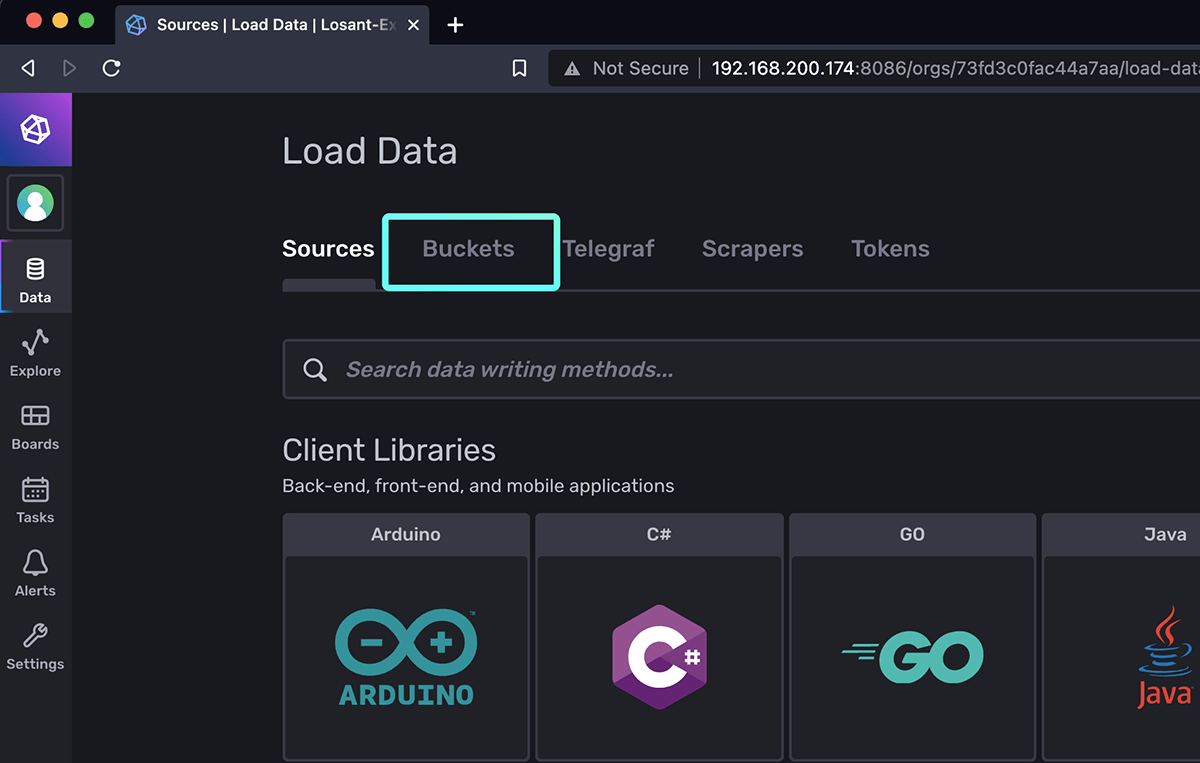The image is a detailed screenshot of a web interface showcasing a data management platform. At the top of the screen, the browser tab includes partially visible labels such as "Sources," "Load Data," and "Locent," before being cut off. The URL in the address bar is highlighted as "Not Secure" and reads "192.168.200.174" followed by additional text in darker gray.

The main section of the webpage prominently displays a title "Load Data" accompanied by several interactive buttons: "Sources," "Buckets" (outlined in a bright blue thin rectangle), "Telegraph," "Scrapers," and "Tokens." Directly beneath this, there is a search bar labeled "Search data writing methods."

Further down, a categorized section lists various resources including "Client Libraries," "Back-end," "Front-end," and "Mobile Applications." Under these categories are icons labeled with programming languages and environments such as Arduino, C#, Go, and Java.

Running vertically along the left side of the interface, there are navigation buttons for "Data," "Explore," "Boards," "Tasks," "Alerts," and "Settings." At the very top of these navigation buttons is a profile icon, presumably providing user account settings and information.